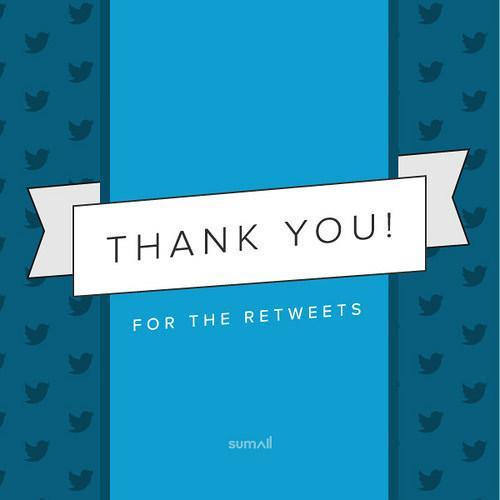The image is a digitally rendered graphic expressing gratitude for retweets. On either side of the image, there are dark blue vertical bands, each occupying about 10% of the width. These bands feature a repeating pattern of bird silhouettes reminiscent of Twitter's old logo. Between these bands, the central portion of the image, which takes up roughly 70%, is a light, bright blue, similar to Twitter's signature color. Across the middle, a white ribbon stretches horizontally, bearing the words "Thank you!" in bold black text. Beneath the ribbon, the phrase "for the retweets" is inscribed in white text. At the bottom center of this blue section, the name "Sumail" appears, likely identifying the individual extending the gratitude. The overall design is simple yet classy, suggesting it was created using digital tools or AI.